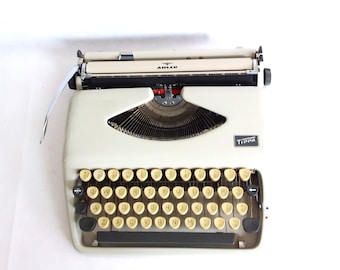The image features an old-styled manual typewriter, reminiscent of models from the early 20th century to the 1970s. The typewriter's body is predominantly off-white with beige and cream-colored accents. Its background transitions from a grayish cream color on the left side to a stark white on the right, creating a striking contrast. The typewriter itself has a metallic frame, with a visible metal piece extending across the top, alongside a black section that provides visual depth.

The individual keys are darker cream or tan, with the metal mechanisms connecting to these keys clearly visible through an opening. This opening also reveals the semicircular arrangement of the metal keystrokes, allowing a glimpse into the inner workings of the machine. There’s notable text on the typewriter, with what appears to be "A-H-E-E-A-D" along the top area and either "TIPPA" or "TEPPA" in the middle section. Additionally, there’s a small black square positioned on the far right.